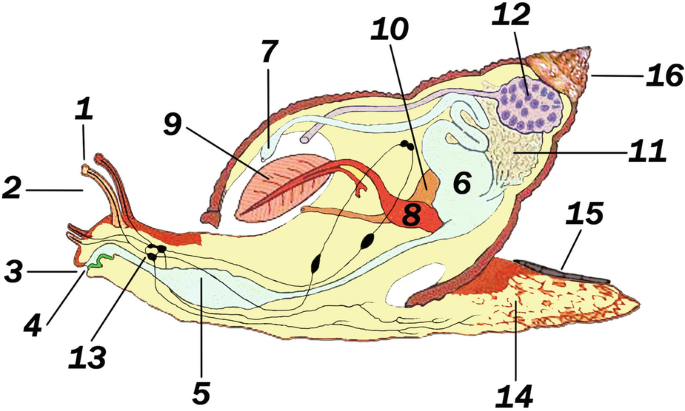This image is a detailed, labeled infographic of a snail, depicting its side profile with an x-ray style view that reveals the internal anatomy. The snail's exterior features hues of yellow, red, and brown, while the internal structures are colored in various shades including purples and reds. The diagram is annotated with numbers ranging from 1 to 16, each pointing to specific parts of the snail without accompanying textual explanations. Key labeled elements include the eyes (1), mouth (3), tongue area (4), a glandular area (13), tail (14), the shell's outer area (16), a purple internal organ (12), an organ resembling a leaf (9), an area presumably the heart (8), and a section that seems like the intestine system (6). The intricate network of organs and connecting tubes typical of a living organism is clearly outlined, presenting a comprehensive view of the snail’s biological structure.